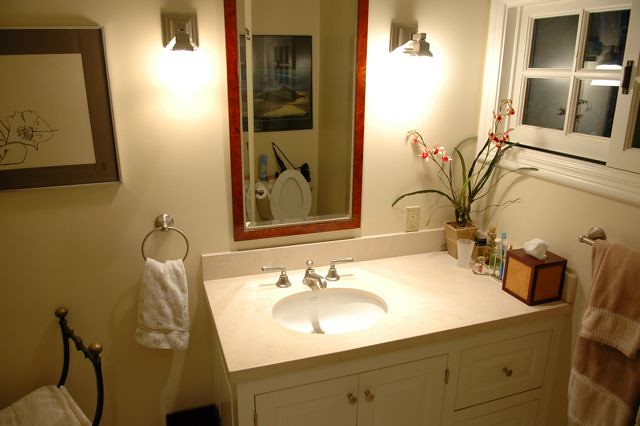The image depicts a well-organized bathroom viewed from the front. Central to the image is a sink set into a tan-colored countertop. The sink features two lever knobs and a silver faucet with a prominent bulbous design on top. Flanking the sink are two white cabinets and a visible drawer on the right, each adorned with gold knobs.

On the far right side of the countertop, there is a wooden box of Kleenex. Just behind the Kleenex box, various items including cups holding toothbrushes and glasses are arranged neatly. Adding a touch of nature, a flower pot sits behind these items, with large vines and blooms extending from it, bringing a hint of greenery to the setting.

Above the sink hangs a mirror bordered with wood. The reflection in the mirror reveals the top of a toilet with its seat raised, and what appears to be either a painting or a television set mounted on the wall above the toilet, adding a decorative as well as functional element to the bathroom space.